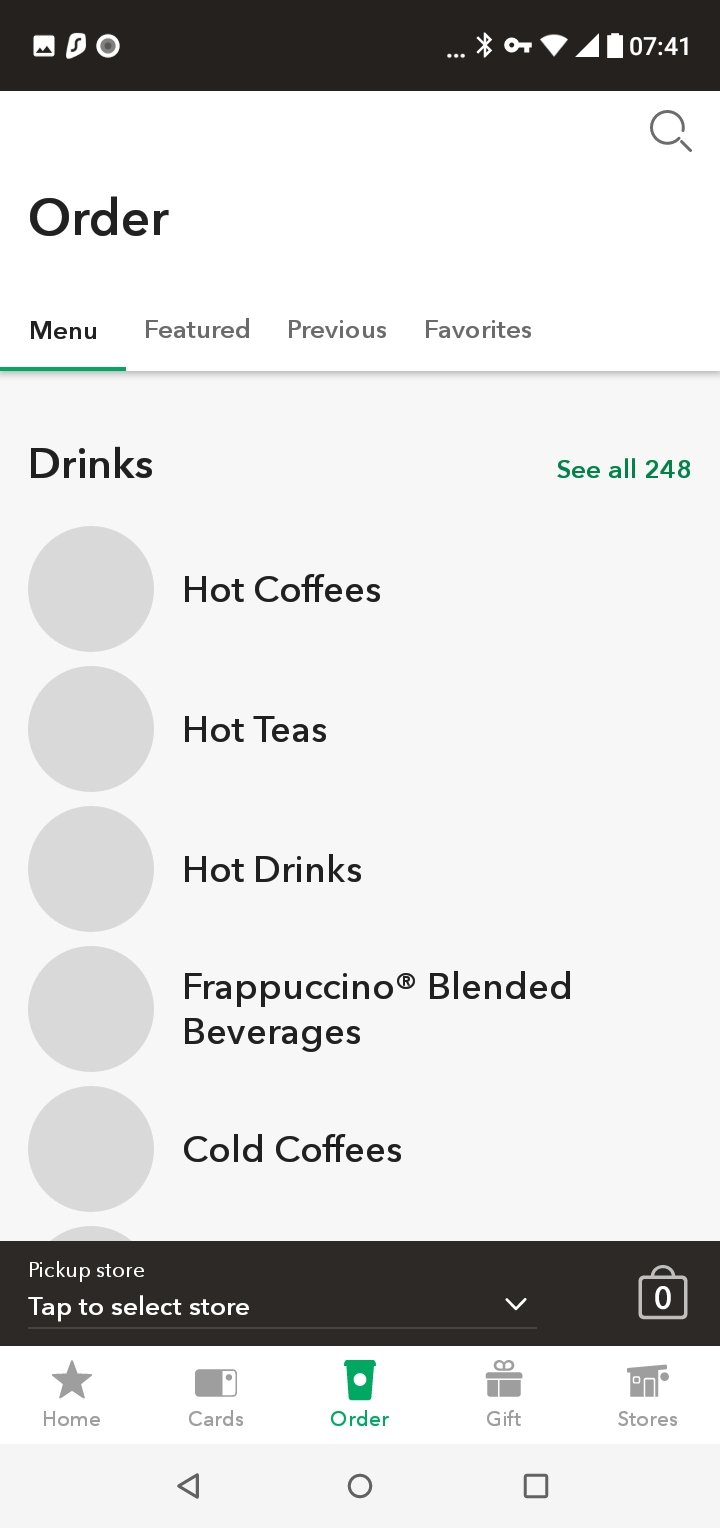The screenshot depicts a smartphone display at 7:41 AM, as indicated by the time in the top right corner, consistent with military time formatting. The battery icon next to the time is fully charged. In the top left, the word "Order" appears in black text. Below this, several navigation tabs are visible, with the "Menu" tab highlighted in green, suggesting the user is currently on this section. 

Adjacent to the "Menu" tab, there are other tabs labeled "Featured," "Previous," and "Favorites." Beneath these tabs, the screen showcases a subsection of the menu titled "Drinks," with an option to "See All 248" drinks detailed in smaller green text on the right side, signifying a large variety. The categories listed under drinks include "Hot Coffee," "Hot Teas," "Hot Drinks," "Frappuccino Blended Beverages," and "Cold Coffees." The clear layout provides an easy-to-navigate interface, revealing the extensive drink options available.